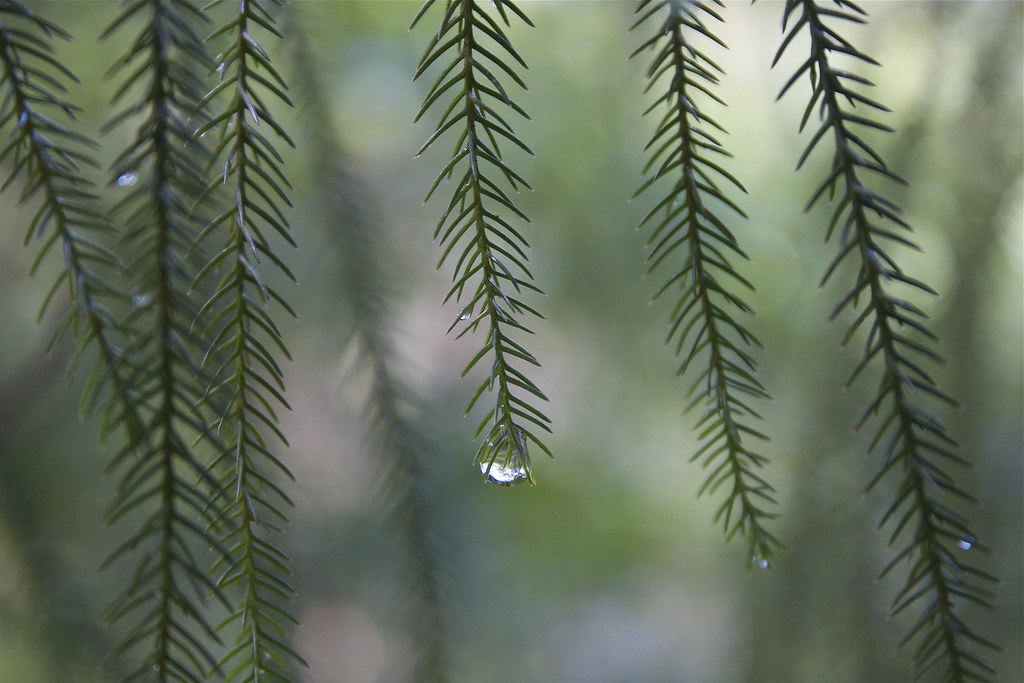This close-up macro photograph showcases six distinct strands of dark green pine needles hanging vertically from an evergreen tree. The focal point of the image is the central needle, which prominently features a large, glistening dewdrop at its tip, reflecting light like a diamond. Smaller dewdrops adorn the other needles, enhancing their delicate, feathered appearance. The background is a soft, blurred mix of additional evergreen branches and subtle hints of white and green, providing a serene and natural backdrop to the sharply focused, rain-kissed pine needles in the foreground.